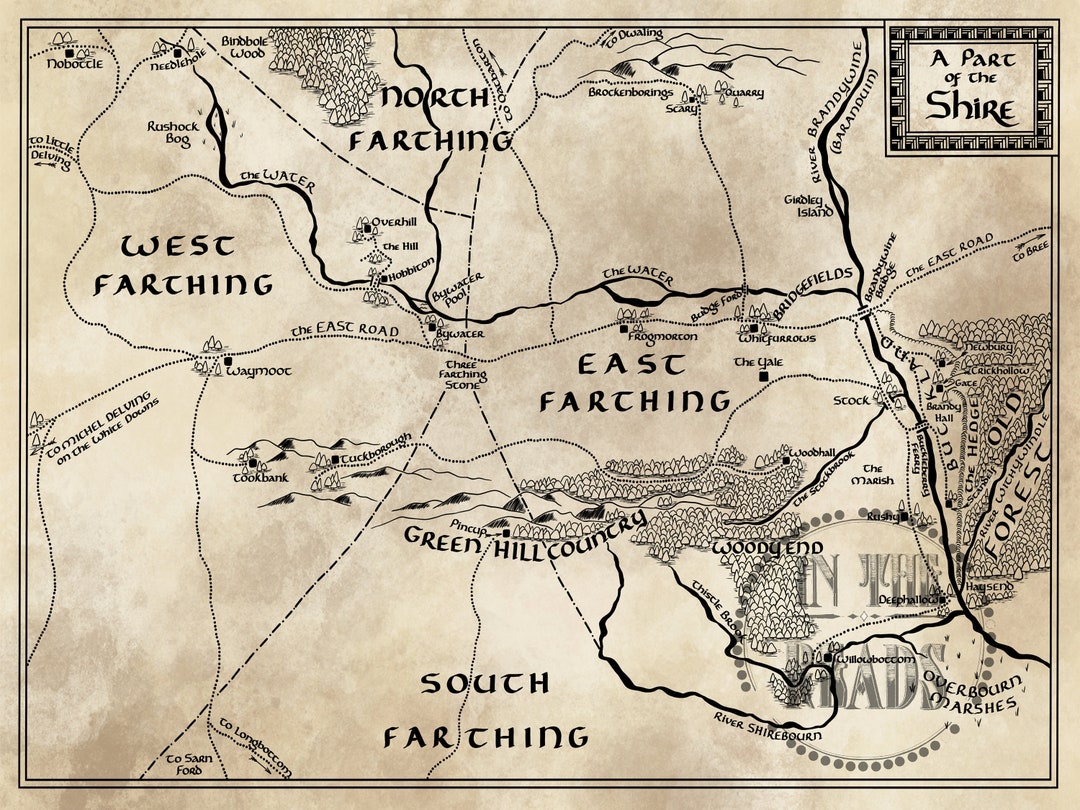The image features an aged, light beige parchment map from the Lord of the Rings universe, specifically depicting a part of the Shire. The map is bordered by a thin black outline, with a small decorative box in the top right corner that reads "a part of the Shire" in elegant, fantasy-style lettering. This corner box is further embellished with a rectangular design made of black squares. 

The map is divided into four quadrants, each labeled with large black text: North Farthing at the top, West Farthing on the left, East Farthing on the right, and South Farthing at the bottom. In the upper central area, locations such as Brockenborings, Scary, and Quarry are marked with charcoal-shaded hills. To the left lies Bindbowl Woods, and to the south of this area is Hobbiton, flanked by The Hill and Underhill. 

The map includes multiple crisscrossing lines representing roads and rivers, with dotted and dashed lines indicating pathways. Distinct regions like Green Hill Country and Woody End are prominently displayed, the latter being depicted with an abstract woodland texture. 

On the bottom right corner of the map is a notable circle watermark with ornate gray text that reads "In the Roads," surrounded by a circle of gray dots. Throughout the map, various symbols denote towns such as Frogmorton, Whitfurrows, and the Old Forest, which is filled with tree symbols, like other wooded areas.